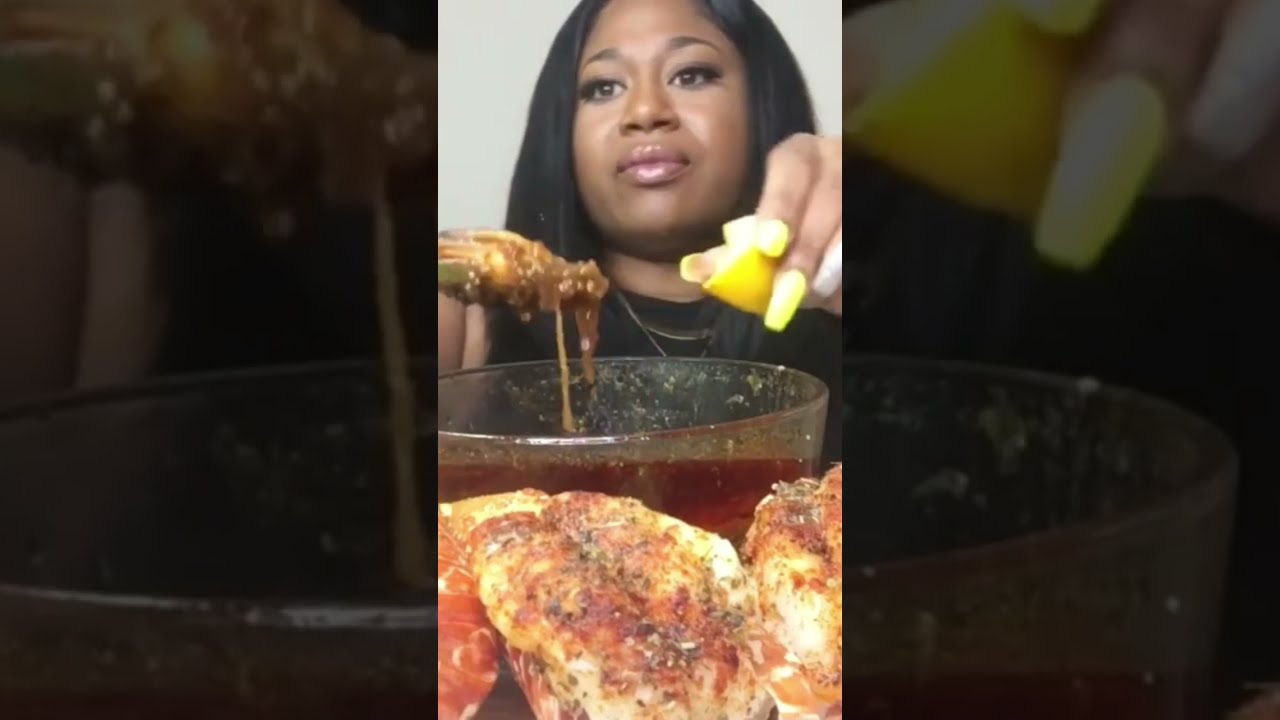In this vertically taken cell phone snapshot, an African American woman with dark, long straight hair and distinctive long yellow fingernails is seen preparing what appears to be a dish involving seasoned meat. The image captures her standing indoors against a light background, possibly indicative of a kitchen setting. In her left hand, she is squeezing a lemon over a large clear glass bowl that contains a sauce, likely a hot sauce or glaze, given the red hue of the liquid. In her right hand, she holds a piece of well-seasoned meat, possibly chicken or seafood, which drips sauce back into the bowl. The foreground prominently features the seasoned meat, hinting at the culinary context of the scene. The woman's facial expression is neutral to slightly disgusted, and she wears a black shirt, focusing intently on the task at hand. This scenario appears like it could be from an Instagram or TikTok reel, emphasizing a moment of food preparation with the smartphone's aspect ratio capturing every detail.